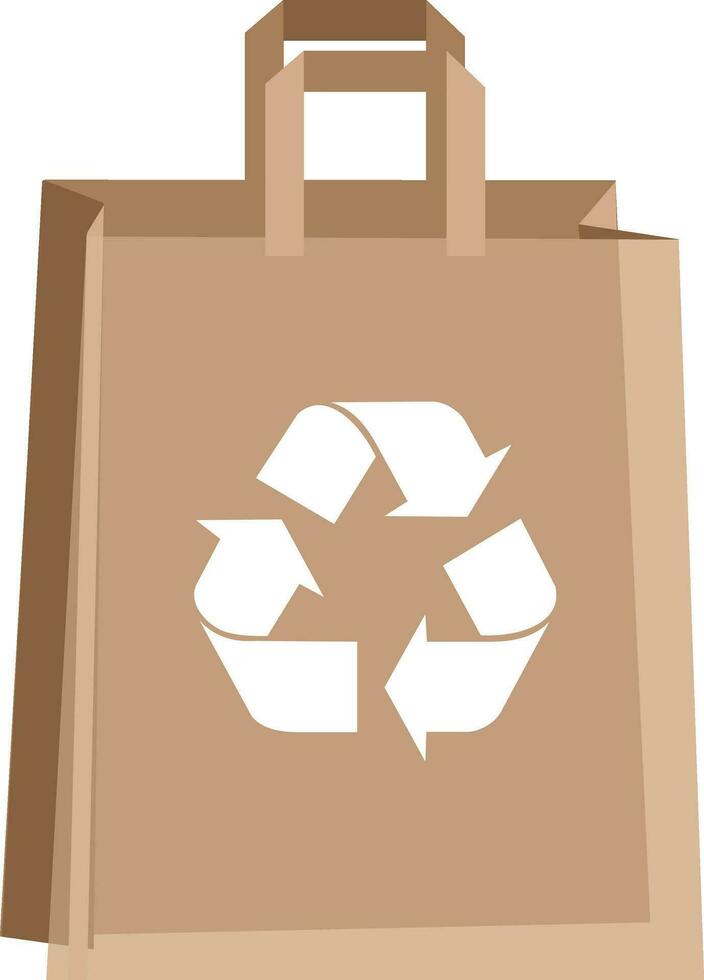The image depicts a detailed, computer-generated clip art of a brown paper bag set against a white background. The bag is standing upright, unfolded, and open, casting shadows that accentuate its folds and creases. It features two paper handles at the top, both standing erect. On the front of the bag, prominently displayed, is the Recycle logo. This logo is composed of three white arrows, each resembling a folded ribbon, arranged to form a continuous triangular loop, pointing towards each other to symbolize recycling. The overall brown hue of the bag is a light shade, and it appears empty, serving as an illustration to encourage reusing and recycling.